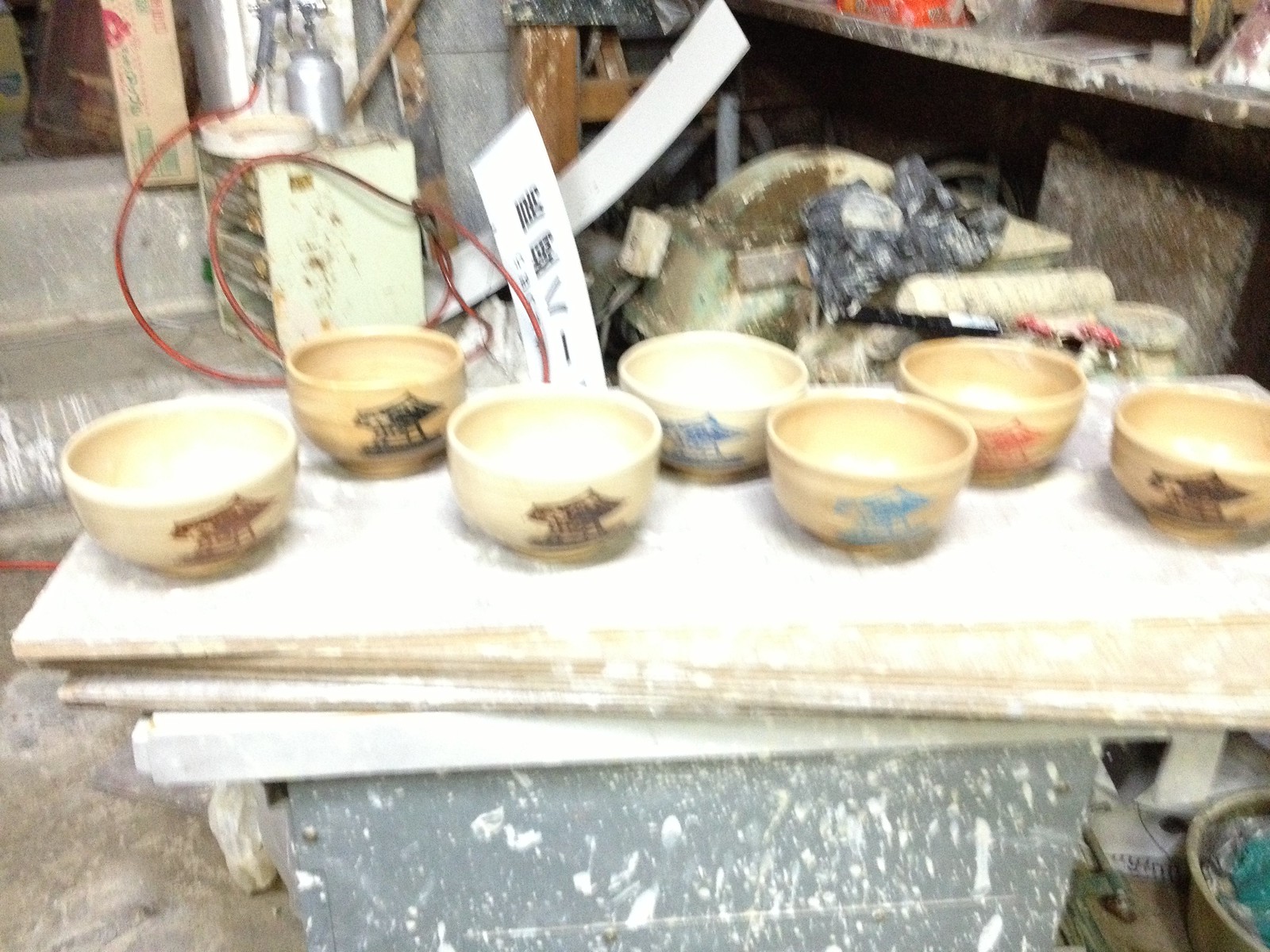This somewhat out-of-focus photograph captures a cluttered workspace dominated by what appears to be a stone table topped with several well-used, wood-stained planks. These planks, perhaps dusted with dried ceramic clay, serve as the base for seven distinct ceramic bowls. Each bowl, finished and fired, features an illustration of a creature—possibly a tiger, wild pig, or an Asian architectural motif in various colors including blue, brown, red, and black. The bowls are arranged with three in the back and four staggered in front.

In the disordered background, a miscellany of items can be seen, including piled plastic bags, large kilns, and shelves scattered with stone-like tools and objects, all seemingly splattered with paint or another dried white substance. The workspace appears to be outdoors or semi-outdoors, given the presence of stone steps and a door leading into another structure at the top left. A white rectangular sign with what looks like Chinese writing adds to the eclectic environment, emphasizing the creative yet chaotic nature of the scene.